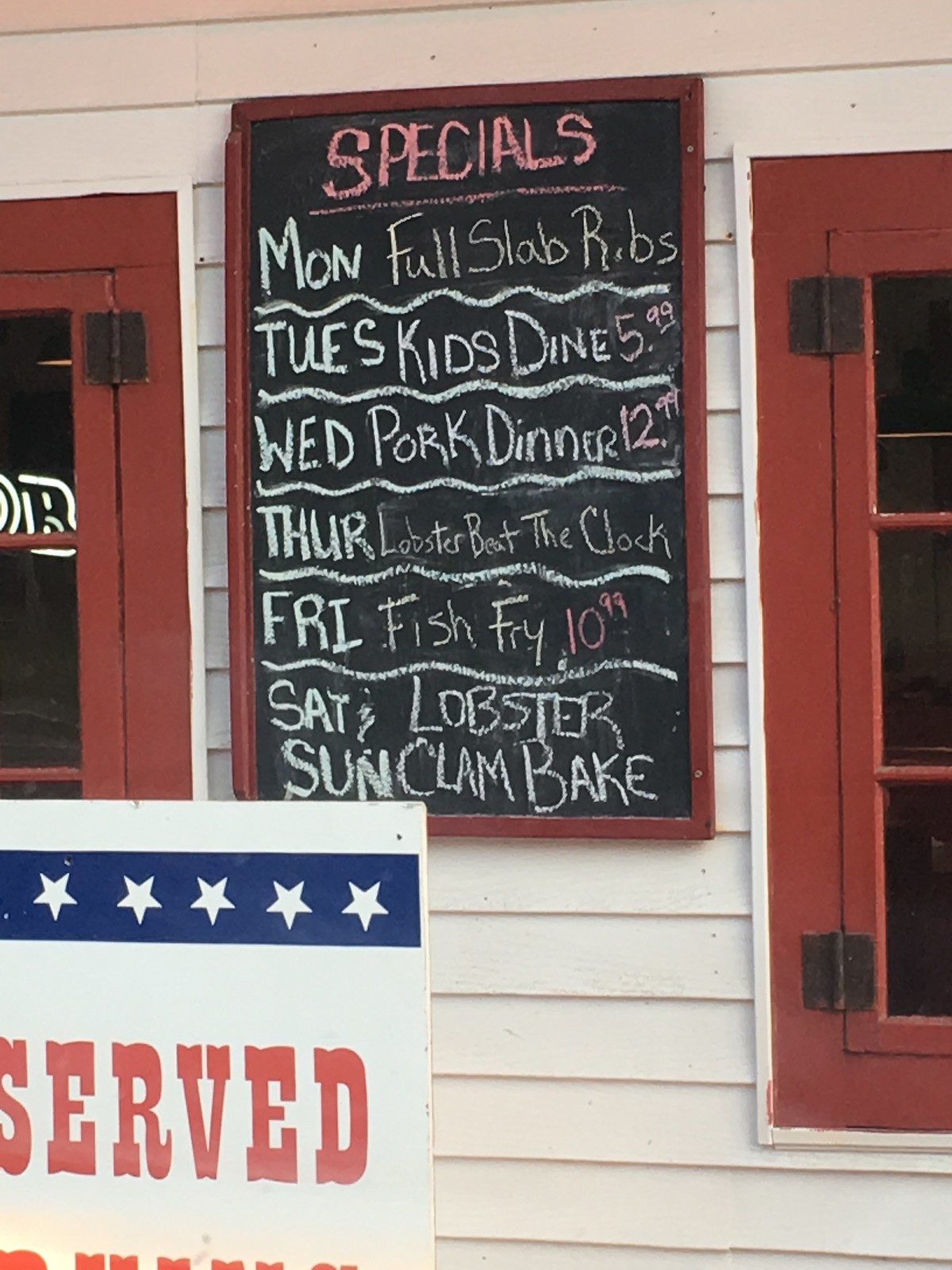Outside a charming New England or Martha's Vineyard café, the exterior is characterized by classic white clapboard siding complemented by striking red window frames and sills. The windows are divided into six sections, each featuring sturdy metallic fittings that add a rugged touch to the otherwise quaint aesthetic. 

Mounted to the side of the café is a chalkboard menu, handwritten with vibrant red and pink chalk. At the top, underlined in pink, the word "Specials" stands out, leading into the daily offerings:

- **Monday:** Full Slab Ribs
- **Tuesday:** Kids Dine for $5.99
- **Wednesday:** Pork Dinner for $12.99
- **Thursday:** Lobster Beat the Clock
- **Friday:** Fish Fry for $10.99
- **Saturday:** Lobster
- **Sunday:** Clam Bake

In the left-hand corner of the image, a portion of a patriotic sign catches the eye. It features a blue stripe adorned with white stars and has red letters below reading "Served," but the remaining red text below is not fully legible.

The scene is completed with the feel of a cozy, community-centered eatery that promises a week of delectable specials in a distinctly American coastal setting.